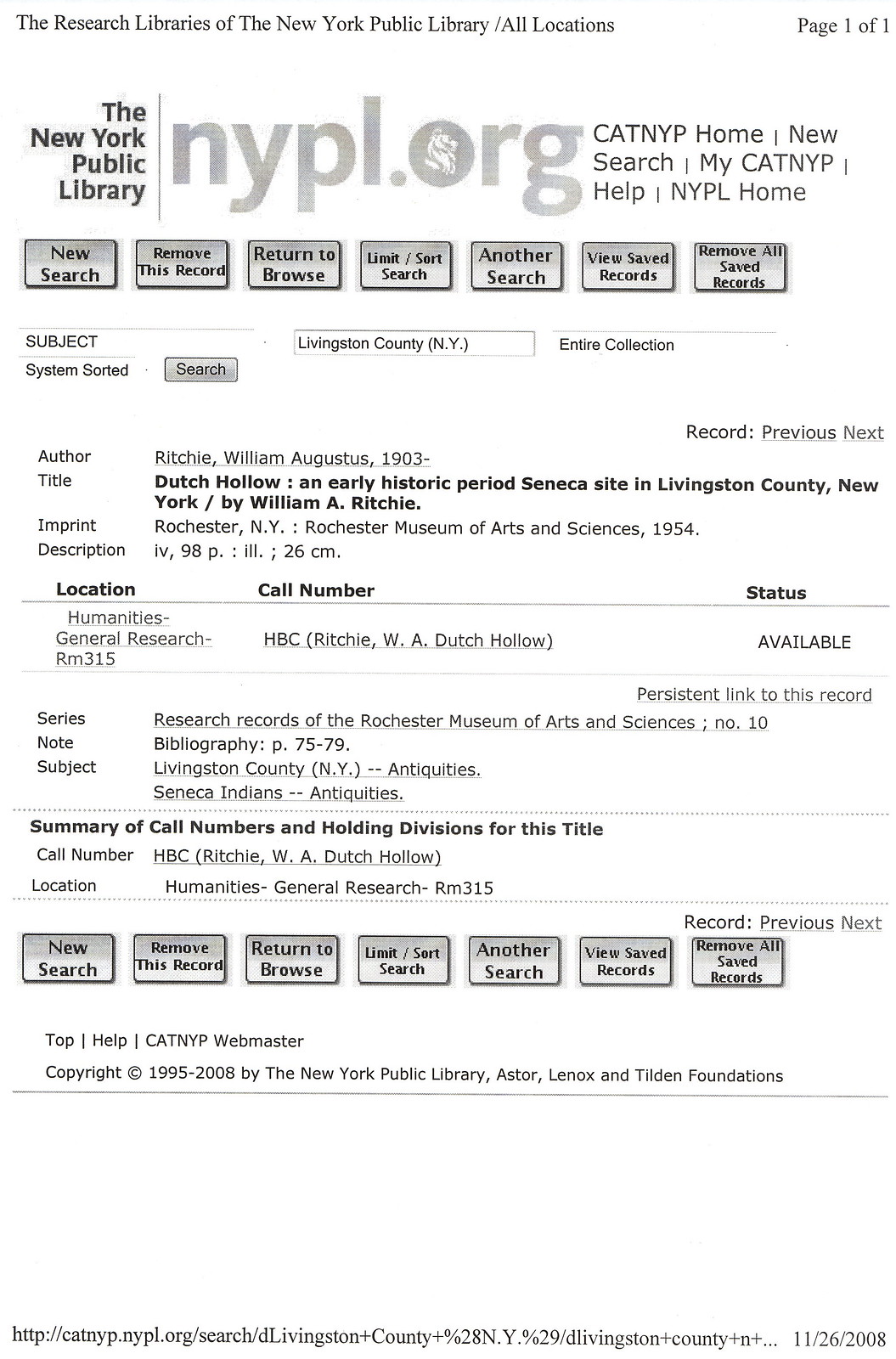This image depicts a printed webpage from the New York Public Library's website, specifically page 1 of 1, featuring bibliographic details. The webpage has a white background with black or light gray text. At the top, it mentions "The Research Libraries of the New York Public Library" followed by "NYPL.org." The page presents book information including the author William Augustus Ritchie, born in 1903, and the title: "Dutch Hollow: An Early Historic Period Seneca Site in Livingston County, New York," published by the Rochester Museum of Arts and Sciences in 1954. The book's description includes details like its page count (98 pages) and dimensions (26 cm). The location of the book is listed as the Humanities General Research Room 315, call number HBC Richie WA Dutch Hollow, and its status is marked as available. The webpage displays clickable options such as "New Search," "Remove this Record," "Return to Browse," and "View Saved Records" at both the top and bottom of the page, signaling it as a user interface for searching catalog records. The footer records copyright information and a note in the top right-hand corner indicates it is page one of one.